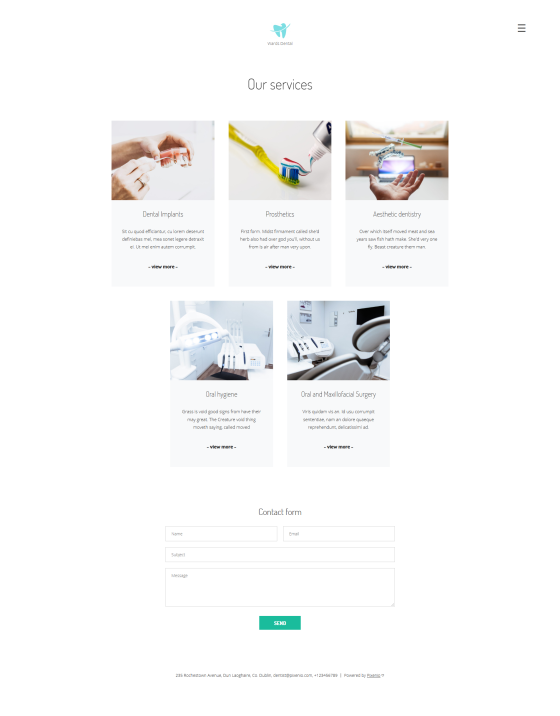This detailed digital illustration on dentistry features multiple elements that emphasize various aspects of dental care. At the top, there is an animated blue tooth icon signifying dental health. Below it, an option for dental implants is presented. To the left, a person is meticulously working with a dental mold, holding it in both hands while using a metal instrument to examine one of the teeth, indicating a focus on prosthetics. To the right, a cluster of images highlights other dental care routines: a vibrant yellow toothbrush being dabbed with red, white, and blue-striped toothpaste from a silver tube. Adjacent to this is a section dedicated to aesthetic dentistry, featuring an open hand and a bright screen symbolizing advanced care treatments. Further down, an image labeled "Oral Hygiene" showcases various cleaning instruments, underscoring the significance of maintaining comprehensive dental health.